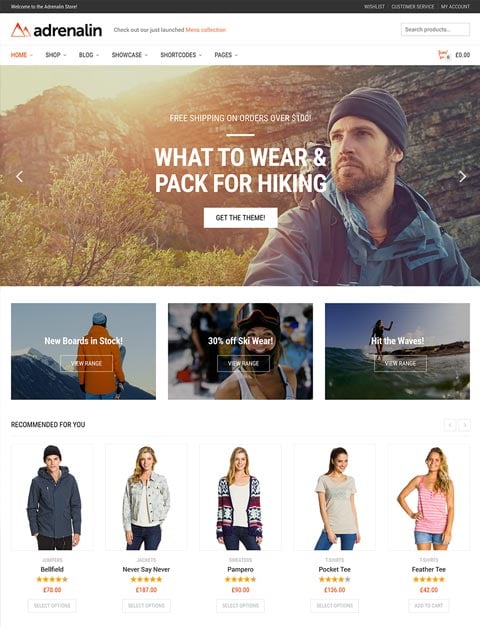The image showcases the website "Adrenaline," formally spelled A-D-R-E-N-A-L-I-N. The homepage features a sleek navigation bar with tabs for Home (highlighted in orange), Shop, Blog, Showcase, Shortcodes, and Pages (all in black, and presumably with drop-down menus). A search box on the right allows users to search for specific products.

At the forefront, there is a visually captivating hero image carousel with left and right navigation arrows. The current image depicts a man poised for a hiking adventure in the mountains. Accompanying the image is a message highlighting the website's offer: "Free shipping on orders over $100" and a guide on "What to Wear and Pack for Hiking."

Beneath this main section are three promotional tiles. The first tile, "New Boards in Stock," features an individual holding a snowboard, suggesting new arrivals in snowboarding gear with a prompt to "View Range." The second tile, "30% Off Ski Wear," depicts a woman dressed in ski attire, enticing visitors with a discount offer on ski wear, again with a "View Range" button. The third tile, "Hit the Waves," shows a woman surfing, encouraging users to explore surfwear via a "View Range" link.

Finally, there is a "Recommended for You" section displaying five more images of individuals, one man and four women, each showcasing different apparel items.